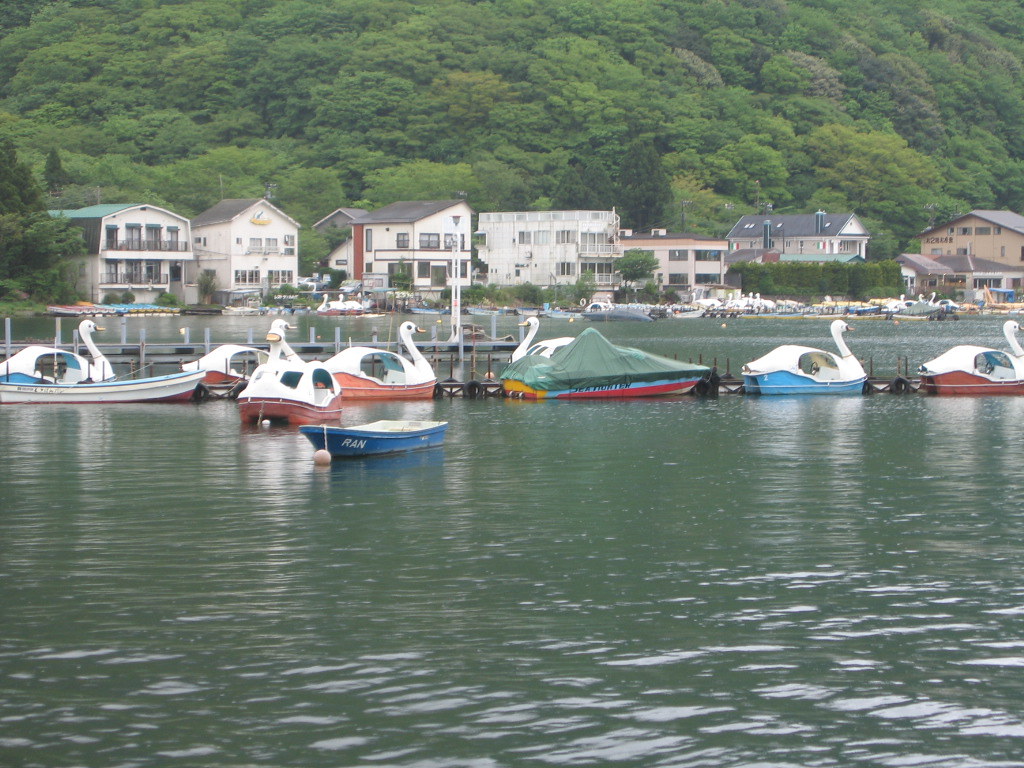This image captures a serene lake scene, where the water takes on an opaque forest green hue. Along the shoreline, a scattering of multiple two-story houses predominantly painted white with black roofs can be seen, with a few exceptions: one house on the far right is light brown with a blackish roof, and another on the far left boasts a distinctive teal roof. The houses overlook the lake, accompanied by docks extending into the water.

The lake itself is dotted with whimsical paddle boats designed to resemble swans. These fiberglass swan boats feature large heads at the front, tapering bodies, and can typically hold two people who steer using a wheel. They are arrayed in various colors, including dark orange and light blue. At least seven swan boats are visible, along with a regular boat that is covered with a green tarp and has a blue and red streak on it. Near these boats, a small black lining is visible.

In the background, a lush, tree-covered hill rises, providing a picturesque backdrop. The overall scene is quiet and tranquil, with no people in sight, under a cloudy sky. An Italian flag hints at the possibility of the location being in Italy or of an Italian influence.